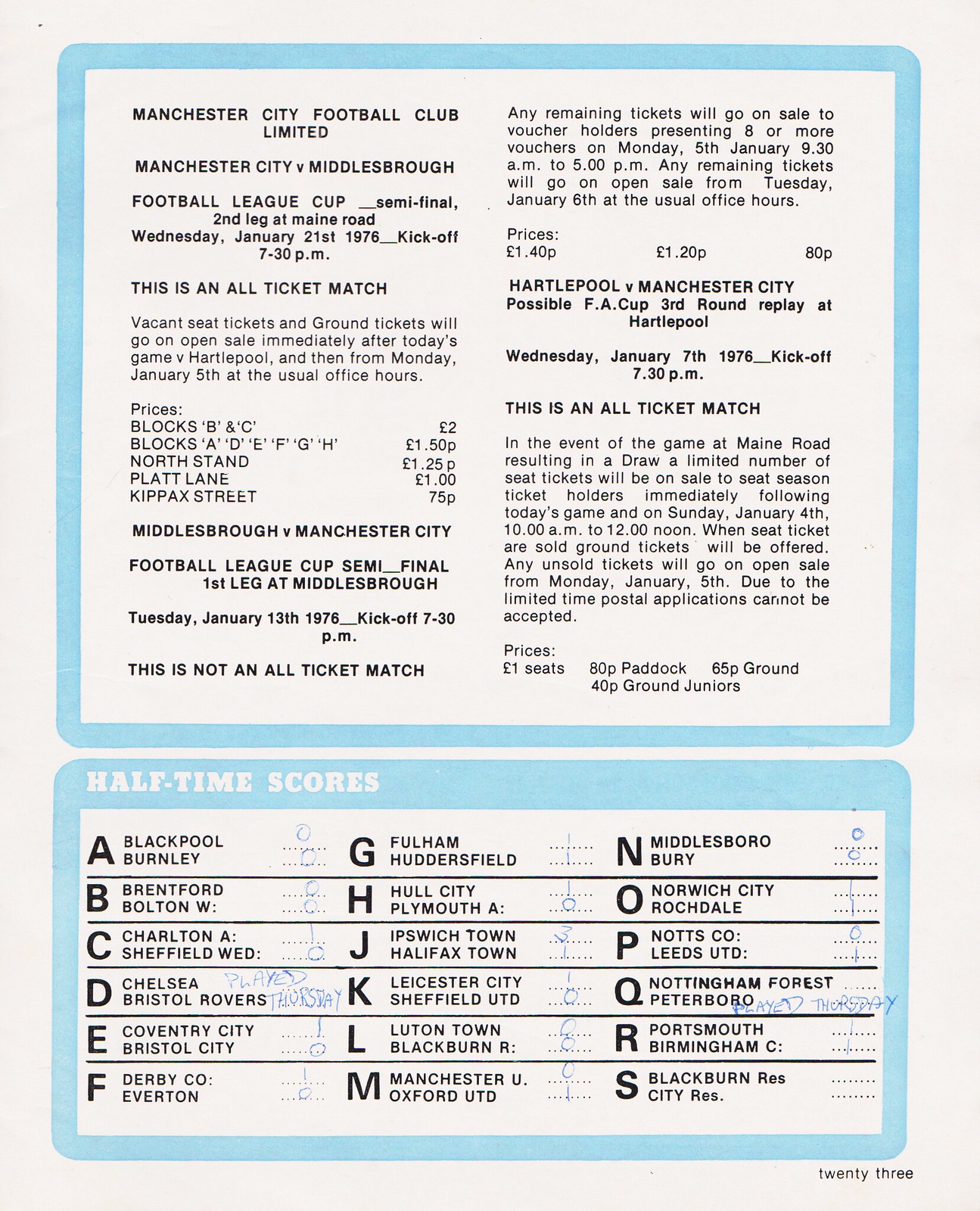The image depicts a page from a 1976 soccer magazine focusing on the Manchester City Football Club. It prominently features details of the Football League Cup semi-final second leg between Manchester City and Middlesbrough, scheduled for Wednesday, January 21st, 1976, with a kickoff at 7:30 p.m. The page displays ticket prices for various stands: Blocks B and C at two pounds, Blocks A, D, E, F, G, and H at 1.50 pounds, the North Stand at 1.25 pounds, Plat Lane at one pound, and Kippax Street at 0.75 pounds. Additionally, there is some content about another match featuring Hartlepool versus Manchester City. The page includes a scoreboard section with half-time scores of several English League games, listing teams such as Blackpool vs. Burnley, Brentford vs. Bolton, and Charlton Athletic vs. Sheffield Wednesday among others, labeled from A to S. This scoreboard section is split into three columns, each containing five matches. Despite the text being small and challenging to read, the publication showcases both historical match details and team scores. The overall look of the page is accented with turquoise borders and is marked as page 33 at the bottom right corner.